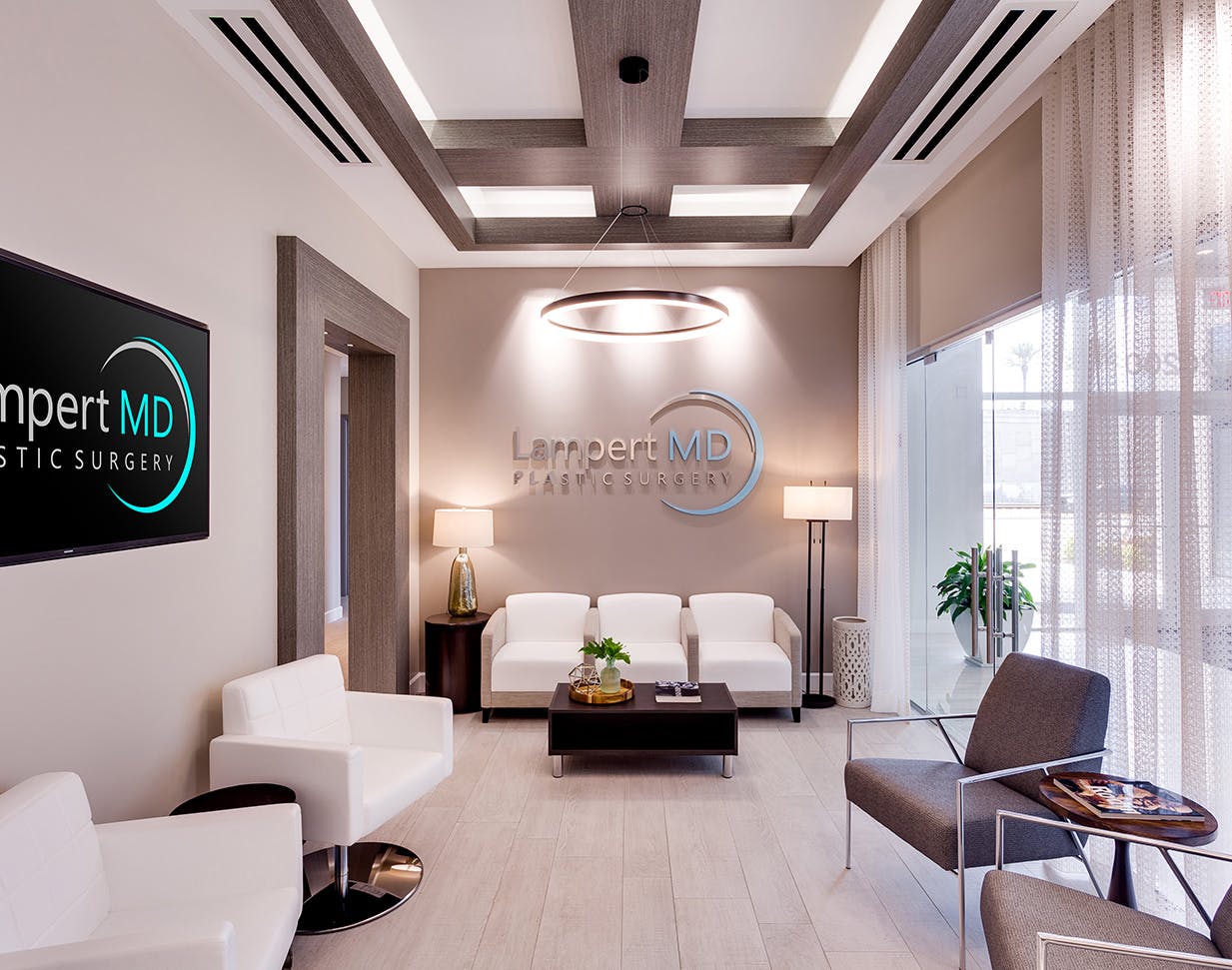The image depicts the waiting room of Lampert MD Plastic Surgery, characterized by a neutral-toned, long, and narrow space with a sophisticated mid-century modern aesthetic. The room is anchored by a deep tan taupe wall at one end, prominently featuring a standout 3D sign of "Lampert MD Plastic Surgery," where "MD" is in blue and "Lampert" is in various shades of tan, encircled by a partial half-circle. 

To the left of this sign, there are two plush white chairs flanking a small side table. The adjacent wall houses a black sign, also indicating the clinic's name. To the right, beneath sheer curtains and a large window, are two brown chairs with an accompanying brown table. Further down the room, a comfortable three-seated white and tan couch sits in front of a coffee table adorned with a plant and a book, flanked by two lamps—one standing and one on an end table.

A TV screen on the left wall mirrors the clinic's logo, contributing to the luxurious feel, underscored by the chandelier overhead that emits a soft halo of light, echoing the circle theme of the logo. The ceiling is detailed with framed dark woodwork, enhancing the room's elegant design. The room, with its modern chrome and gray upholstered furniture, together with the strategic placement of side tables possibly holding magazines, exudes a high-end atmosphere appropriate for a plastic surgery clinic where aesthetics and comfort are paramount.